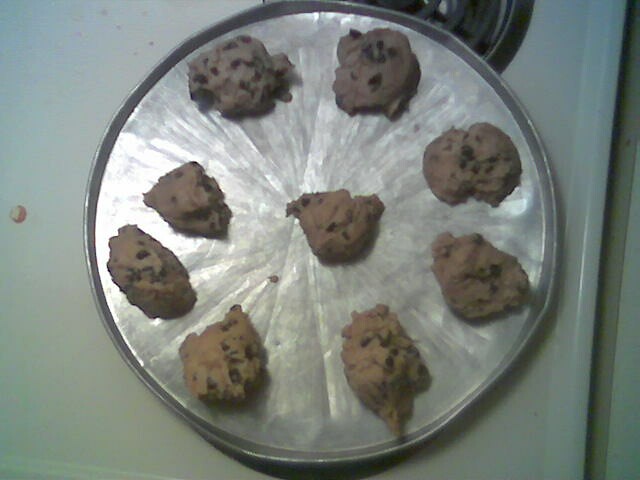This image captures a silver, round baking tray that appears slightly dented and aged, resting atop a white stove. The well-used, shiny pan is arranged with nine uneven blobs of chocolate chip cookie dough; eight form a circle around the edge, and one is positioned in the center. The dough is unbaked, with a mix of brown and dark chocolate chips visible in each mound. In the top part of the image, a black circular burner from the electric stove can be seen, while the right side of the photo shows the edge of a dark object, adding to the kitchen setting. A hint of a red object is also visible on the left, juxtaposing against the white background.